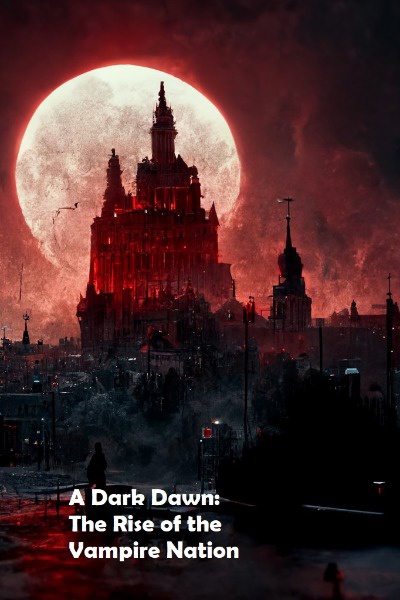The image is a computer-generated piece of artwork in portrait orientation, likely resembling a poster or book cover. It depicts a misty, fog-filled night scene. A dark, silhouetted city occupies the foreground, while an imposing, deep red castle with towering spires dominates the center. Looming behind the castle is a large, slightly red-tinted full moon, which casts an eerie glow over the scenery. Red smoke or mist rises ominously into the dark sky, enhancing the gothic atmosphere. Towards the bottom of the image, a dark, silhouetted figure stands with their back to the viewer, gazing into the enigmatic city. In white text, positioned above the figure, the image bears the title, "A Dark Dawn: The Rise of the Vampire Nation."